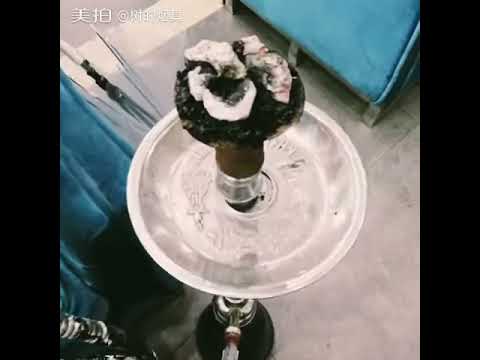This grainy, possibly pixelated image captures an overhead view of a large hookah pipe, centered prominently on a hard, gray concrete or tiled floor. The hookah features a black base, a hose extending from it, and a plate at the top containing what looks like tobacco, crowned with a few rocks, giving the top a bulbous shape with a small cylinder stick. The pipe's midsection is silver, black, and brown with a hint of white at the top, possibly from the tobacco being smoked. Framing the scene, the image includes two light blue couches with silver legs, partially visible on the left and right sides. A black border suggests the aspect ratio of older TV screens, and text in an unidentifiable Asian language appears in the top left corner, along with a watermark. The setting resembles a hookah lounge, albeit viewed through a low-quality screen capture.